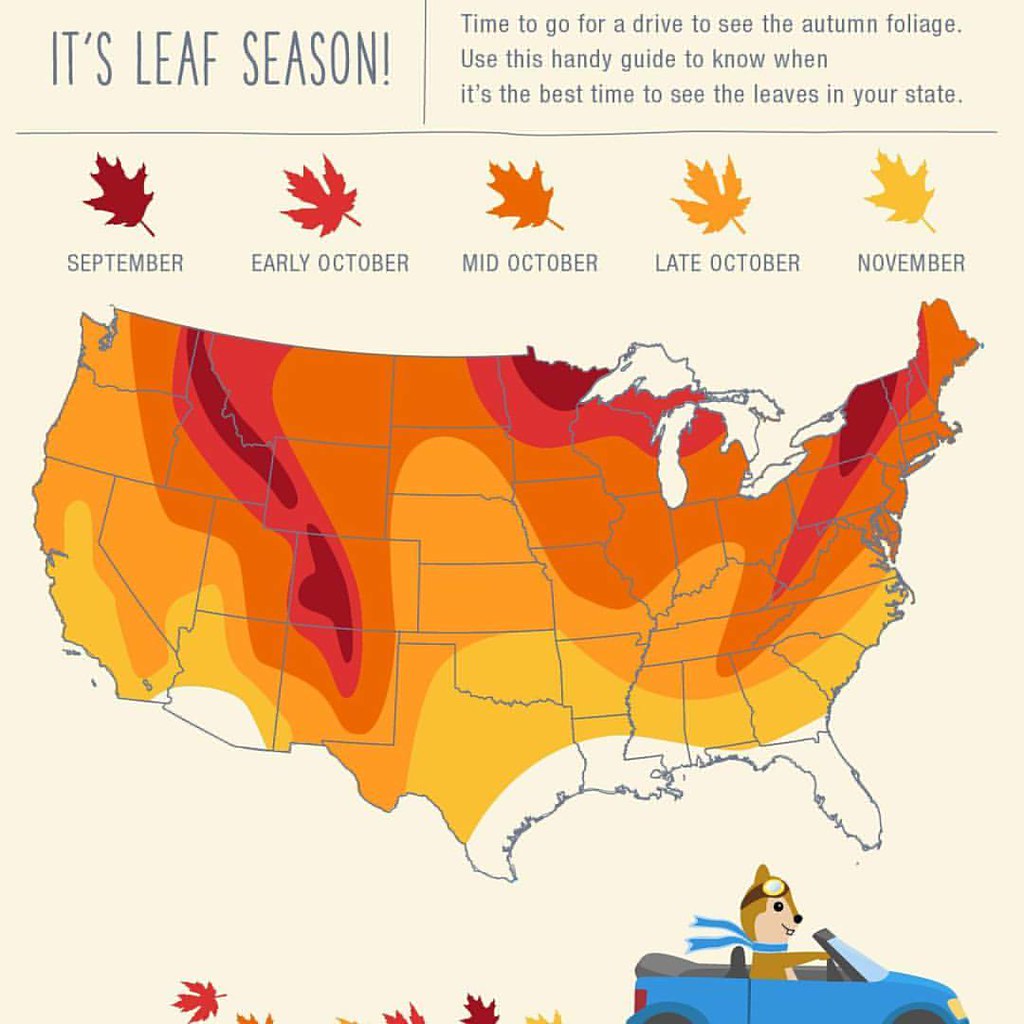The image is an informative advertisement for leaf season across the United States. Centered in the middle is a detailed map of the U.S., serving as a guide to the best times to see autumn foliage in each state. Above the map, various colored leaves indicate the prime viewing months: a very dark red leaf for September, red for early October, dark orange for mid-October, orange for late October, and yellow for November. The text at the top reads: "It's leaf season! Time to go for a drive to see the autumn foliage. Use this handy guide to know when it's the best time to see the leaves in your state." 

In the bottom right corner, a whimsical touch is added with a tan and brown squirrel wearing a matching blue scarf, driving a blue car with a black interior. The squirrel leaves a playful trail of leaves behind, almost like exhaust, enhancing the autumnal theme. The background of the picture is a tan color, and the text is written in a dark blue, almost slate gray, font. This charming and practical image blends the fun of a fall drive with the educational aspects of leaf peeping for all U.S. states.